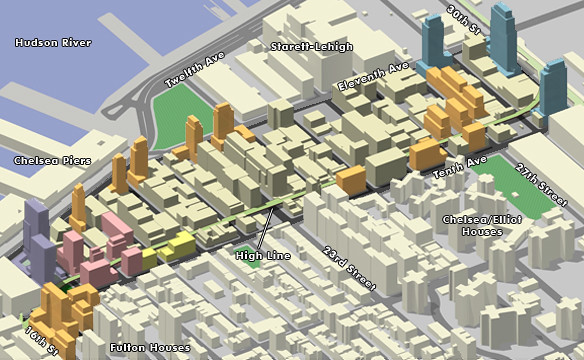This detailed aerial digital map showcases a cityscape with a Lego-like, plasticky appearance, featuring various colored buildings of different heights. In the upper left corner, there's the Hudson River marked in blue, with 'Chelsea Piers' highlighted nearby. The map spans out to show an intricate network of streets, including 12th Avenue, 11th Avenue, and 30th Street at the top, and 16th Street and 23rd Street towards the central and lower left areas. Prominent structures and neighborhoods such as the Fulton Houses and Chelsea/Elliot Houses are labeled, with Fulton Houses near 16th Street and Chelsea/Elliot Houses closer to 10th Avenue and 27th Street. The 'High Line' is marked centrally. The buildings vary in color—white, orange, blue, purple, and light blue—with some depicted as taller than others, contributing to the map's 3D blocky aesthetic that resembles a digital blueprint.